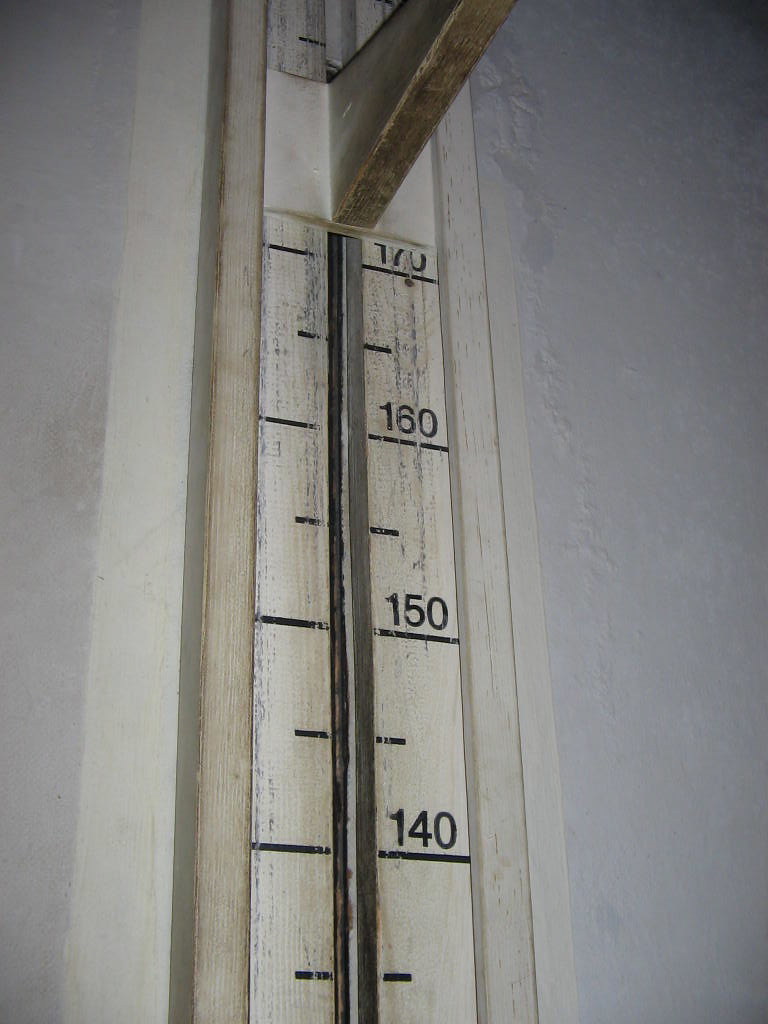This photograph captures a vintage vertical height measuring device, typically found in a doctor's office for measuring patients' heights. The device is mounted on a slightly gray-toned white wall, with shadows creating darker patches in the upper corners. Along the right side of the device, the wall exhibits light texturing, indicating an uneven application of drywall plaster.

The measuring device itself is white but shows significant signs of age and wear. Yellowing and gray vertical scuff marks trace where the measuring piece has been frequently moved up and down. Positioned at the top of the photograph is the measuring slider, a triangular-shaped wedge, which can be manually adjusted. The handle of the slider is noticeably brown from accumulated grime.

The measuring piece is currently set just above the 170 cm mark, with additional visible markers at 160, 150, and 140 cm, descending from top to bottom. The central black groove track of the slider features horizontal bars extending to both sides, with the numerical measurements aligned to the right. Each number is marked with a wide line, and there is a narrower line at the halfway point between each numeral, providing precise measurement intervals.